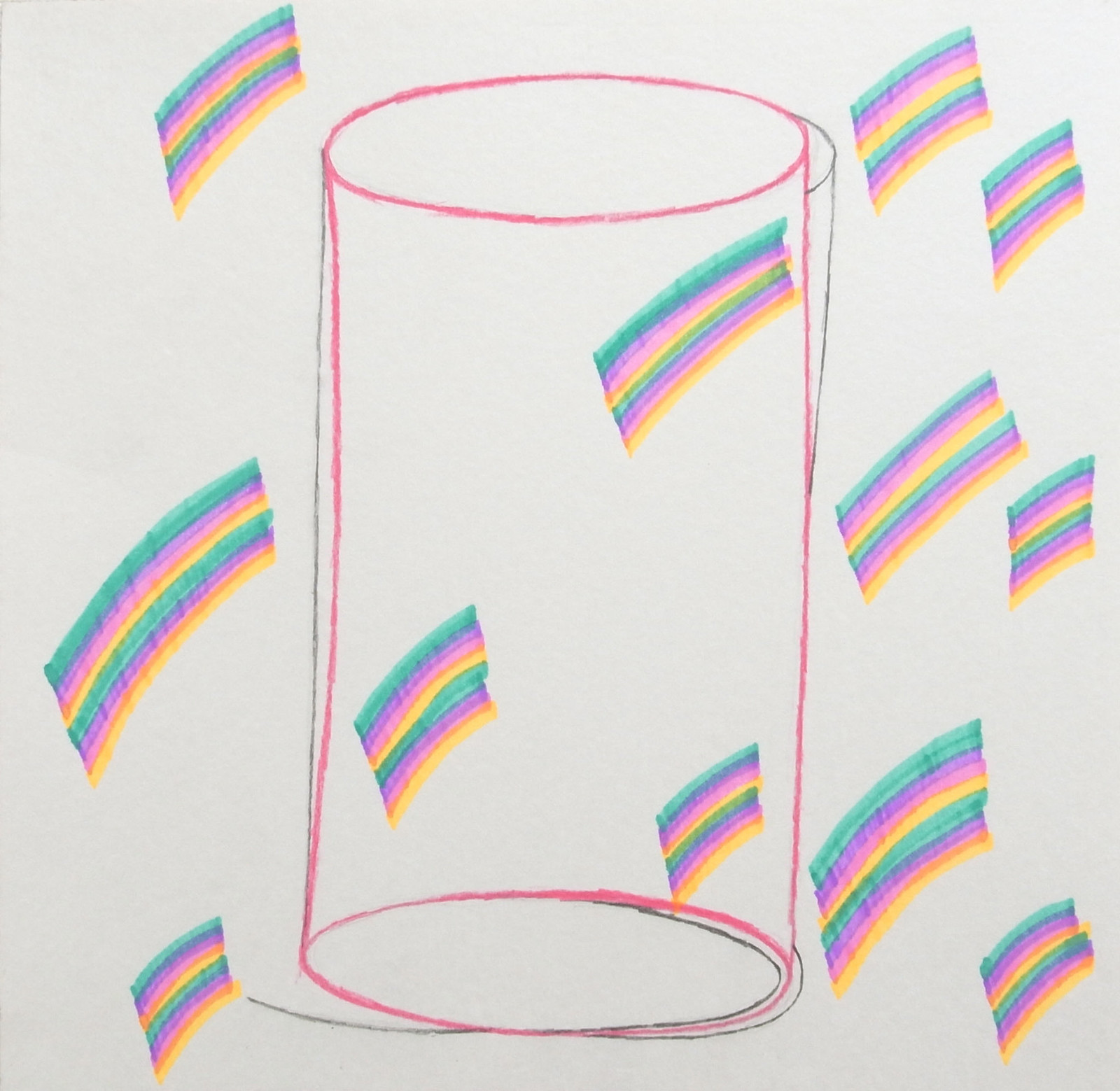This detailed drawing on white construction paper showcases a 3D cylindrical vase centrally positioned. The vase is outlined in red with a three-dimensional effect, enhanced by an additional black outline behind it, giving it depth. The cylindrical shape is emphasized by its tube-like appearance with ovals at the top and bottom, connected by straight vertical lines. Surrounding and partially inside the vase are numerous small, curved strips resembling mini rainbows. These rainbows are meticulously colored in a repeating pattern of green, purple, pink, yellow, green, purple, pink, yellow, and possibly orange. They are strategically placed across the page, with several on each side and three inside the cylinder, creating a whimsical and colorful spread throughout the artwork.